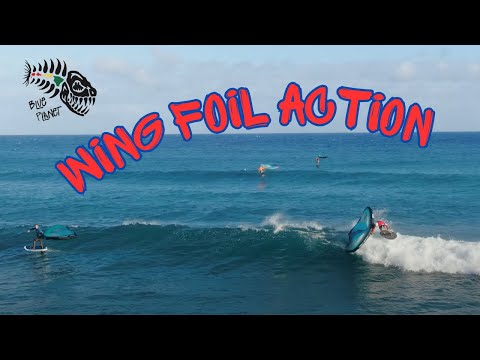This dynamic photograph captures a lively scene of wing foiling and surfing action on the ocean. In the foreground, a man wearing a red shirt skillfully rides a gray skateboard-like board on a white wave, maneuvering a blue wing-like kite above him. To the bottom left, another man, clad in a teal light blue shirt, balances on a white and blue surfboard, holding a similarly colored kite behind him. Further in the background, two more figures, one clearly marked in orange and another barely visible, engage in the same exhilarating sport. Bright red text boldly across the image declares "Wing Foil Action," enhancing the energetic vibe of the scene. In the top left corner, an artistic skeleton of a fish with a rainbow-colored spine is drawn next to the inscription "Blue Planet," adding a unique and colorful touch to the photograph.